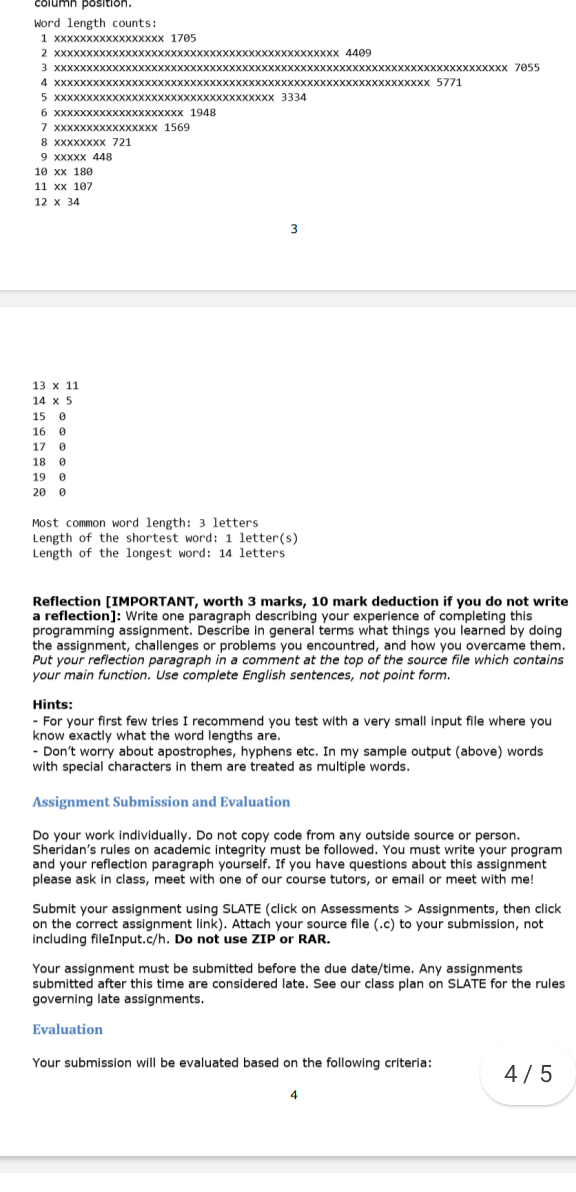In the image, we are looking at a screenshot set against a white background featuring an organized layout of textual information. In the upper left corner, there is the heading "Column Position" written in black text. Beneath it, the text "Word Length Counts" is displayed. Following this, a series of numbers ranging from 1 to 12 are listed vertically down the page. Just below these numbers, a gray line signifies a page break. Continuing from the break, the numbers 13 through 20 are subsequently listed. Underneath these numbers, the text reads "Most Common Word Length: three letters." Further down, it states "Length of the Shortest Word: one letter" and "Length of the Longest Word: 14 letters." At the bottom, in bold black text, the word "Reflection" is prominently displayed, followed by "Important, worth 3 marks." It also includes a warning: "10 mark deduction if you do not write a reflection." The instructions then dictate: "Write one paragraph describing your experience of completing this programming assignment. Describe in general terms what things you learned by doing the assignment, challenges or problems you encountered, and how you overcame them."